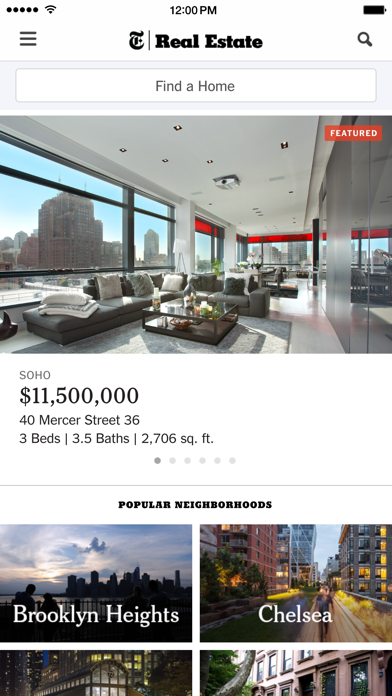This image captures a screenshot, likely from a smartphone or a tablet, given the visible battery icon, wireless signal indicators, and the time displayed as 12 p.m. Thematically, the page features a predominantly white background with black or grey text and several images. At the top, the page is labeled "Real Estate," accompanied by an icon to the left and a magnifying glass on the right.

Below this header lies a search box labeled "Find a Home," inviting users to type in their query. Directly beneath the search box, an attractive image of a property dominates the view. This featured property is an apartment located in Soho, listed for a staggering $11,500,000. The listing details reveal the address as 40 Mercer Street, unit 36, featuring three bedrooms, 3.5 bathrooms, and a spacious 2,706 square feet.

Further down, we encounter a section titled "Popular Neighborhoods," highlighting areas such as Brooklyn Heights and Chelsea. Below this section are additional images of properties, though the accompanying text is not fully visible.

The layout suggests this is a website or application designed for real estate search, currently focused on the New York area. Visual elements are thoughtfully presented with clear black and grey text, punctuated by vibrant, high-quality images. 

The featured property in Soho is showcased with a prominent 'Featured' logo, emphasizing its luxurious appeal. The imagery depicts a modern, elegant apartment with white walls, white flooring, and grey couches. Sunlight floods the space through sizable glass windows, offering views of surrounding buildings, enhancing the upscale aesthetic and confirming the high price tag.